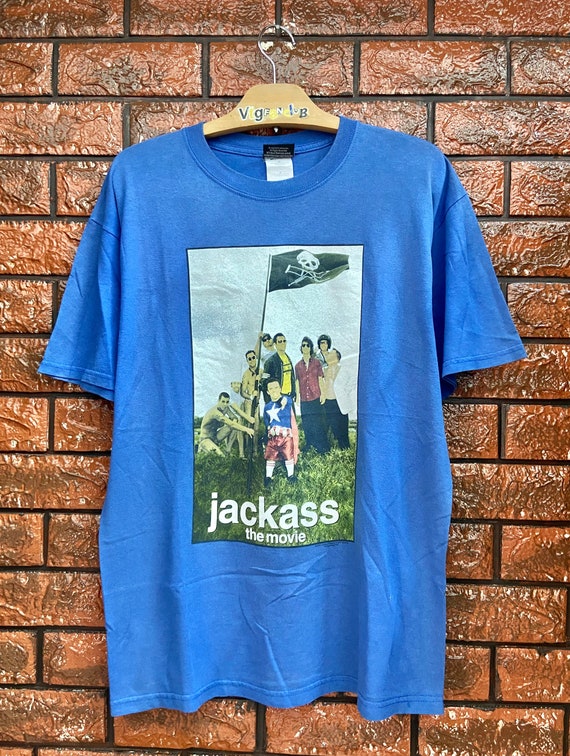This digital photograph captures a blue, short-sleeved t-shirt hanging on a wooden coat hanger against a red brick wall. The light brown hanger is suspended close to the top center of the image by a silver metal hook. The t-shirt features some wrinkles, prominently in the chest area, where a detailed image is printed. This image depicts a group of men standing around a pole adorned with a skull and crossbones pirate flag. Below this graphic, the t-shirt bears the text "Jackass the Movie" in white letters. The composition exhibits a color palette that includes red, brown, yellow, black, blue, green, and white.